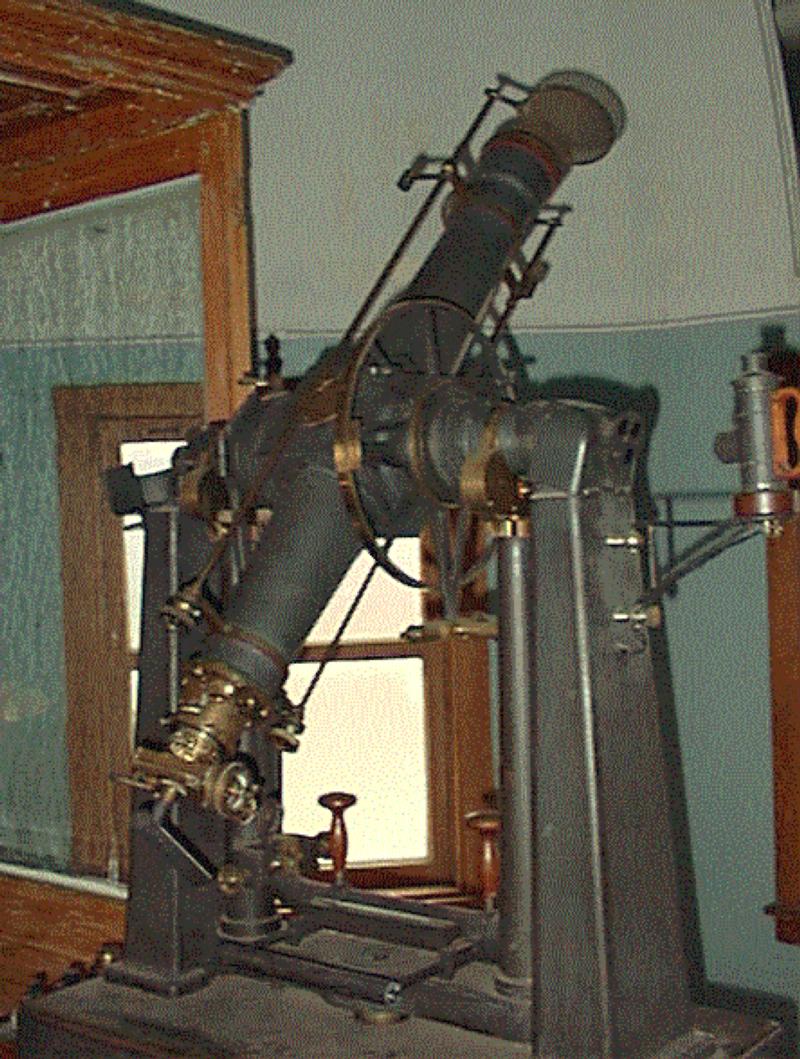The image features a large, old-timey machine, centrally positioned and taking up most of the space. The setting is an old building with wooden ceilings, a hardwood floor in a dark brown shade, and a window framed in dark wood, suggesting a room that possibly could be someone's tool room or a section in a museum. The walls are painted in light blue and white.

The machine itself resembles an early 20th-century observatory telescope or possibly a large microscope, hinting at its historical significance. It's crafted from black metal with brass and copper levers, gears, and a wheel on the side, indicating it can rotate. Dominating the middle of the machine is a big gray cylinder supported by two gray pillars. There is also a cylindrical release or steam valve on one side.

The equipment appears to be dusty, implying it hasn't been used in a long time and is possibly a display piece. The colors in the image range from brown and gray to green, black, and white. The background elements, including the wooden ceilings, walls, and window, add to the antique charm of the scene.